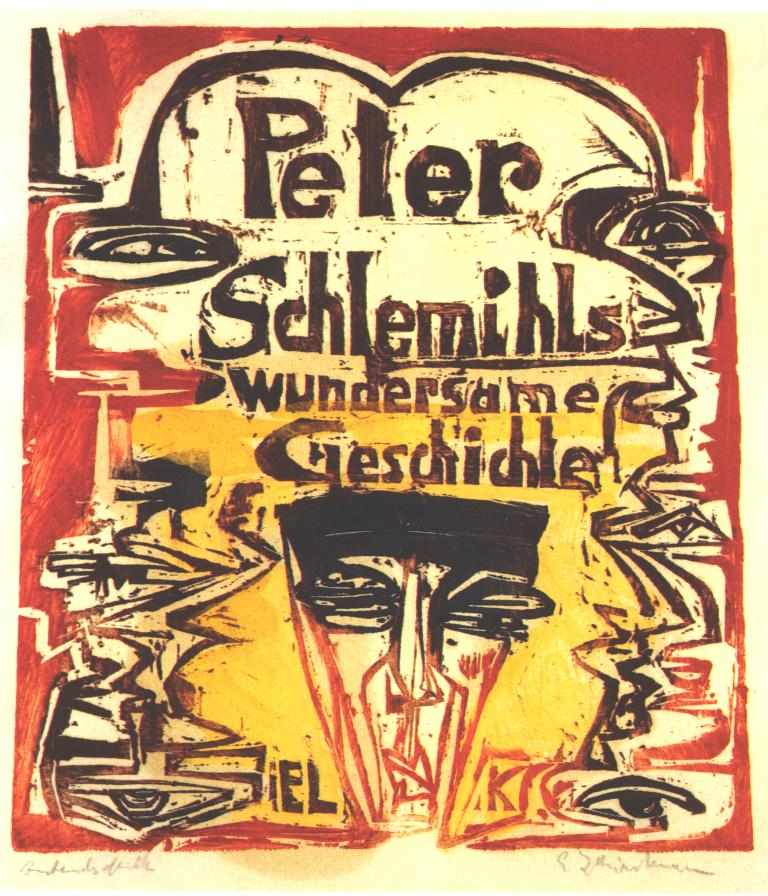The image is a vibrant and abstract poster predominantly featuring a palette of beige, yellow, and red backgrounds. At the top, in bold black letters, it reads "Peter Schlemihl's Wundersame Geschichte," indicating a German text. Surrounding the central text, there are additional decorative letters "E-L" and "K" towards the bottom. The poster features a prominent face in the lower middle, shaped like a pizza slice and outlined in red, with black sunglasses and a black hat, giving the face an abstract wooden chiselled appearance. The facial features include black eyes and abstract red details. Positioned around the face and text are several black squiggles and designs, including rotated black number threes and black eye-like shapes near the top corners and lower right-hand corner. The overall background transitions from beige at the top to yellow in the middle, with red edging around the borders.